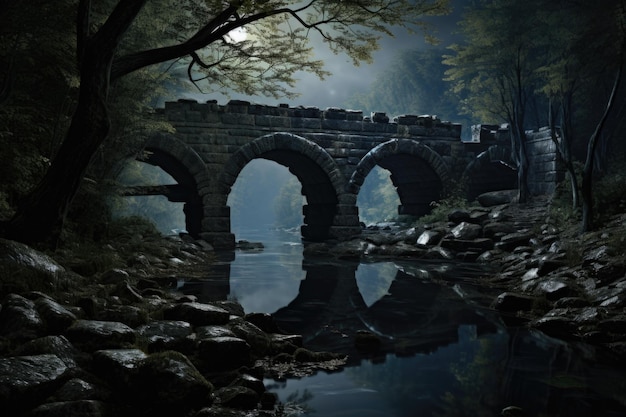In this hauntingly beautiful, photorealistic painting of a moonlit night, a stone bridge stretches majestically across a dark river or stream in the midst of a dense forest. The bridge features four archways, their reflections faintly visible in the tranquil, inky waters below. A crenellated top crowns the bridge, adding a regal touch to its robust stone construction. The scene is illuminated by a mist-shrouded moon positioned in the center left, casting a soft, foggy glow over the landscape. On either side of the bridge, rocky shores frame the water, with trees dotting the edges and extending into the distance. To the left, a tree leans gracefully over the water, contributing to the serene, almost magical atmosphere. Stones and boulders strewn along the banks add texture to the composition, while the forest beyond the bridge stretches into the night, wrapping the scene in natural splendor.